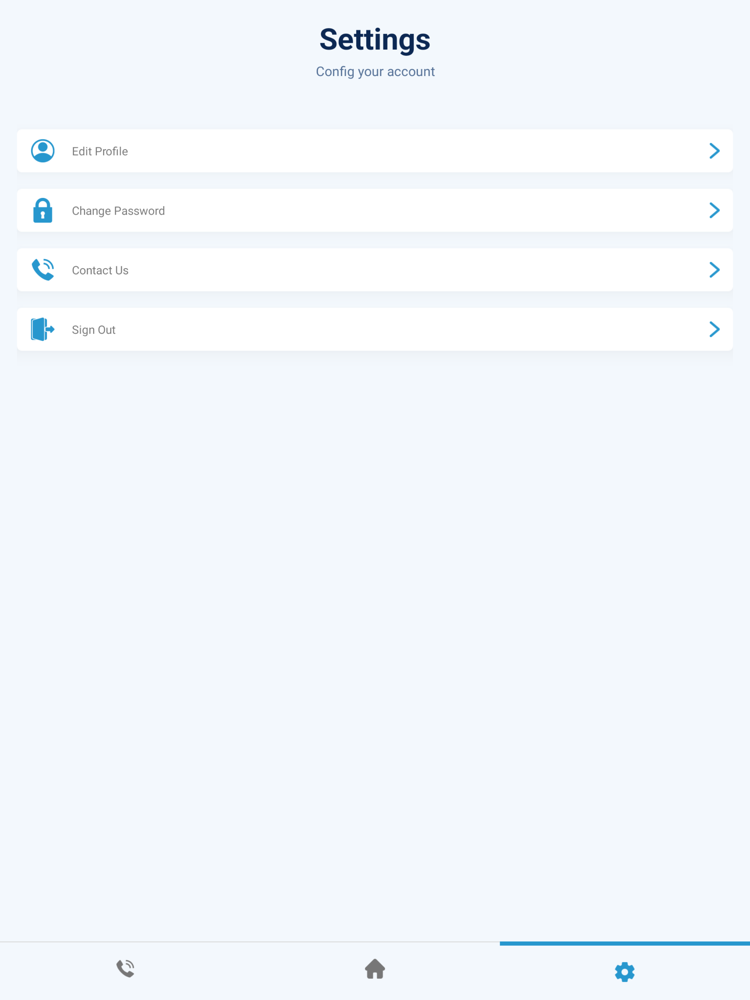This vertical rectangular image features a light blue and grayish background. At the top center, the word "Settings" is prominently displayed in black font. Directly below this, the text "Config Your Account" is written. On the far left side of the page, several icons are arranged in a list:

1. A circular icon with a blue image depicting a person's head and shoulders, labeled "Edit Profile."
2. Below it, an icon of a blue padlock with the text "Change Password" to its right.
3. Further down, an icon of a ringing telephone accompanied by the text "Contact Us."
4. Lastly, an icon of a box or door with an arrow pointing to the right, labeled "Sign Out."

The middle section of the page contains significant blank space without any images or text.

At the very bottom of the page, three icons are aligned horizontally:
- On the far bottom left corner, there is another icon of a ringing telephone.
- In the center bottom, an icon depicting a house.
- Finally, on the far bottom right corner, an icon of a gear.

This organized layout provides a clear and concise navigation structure for users to interact with various settings options.